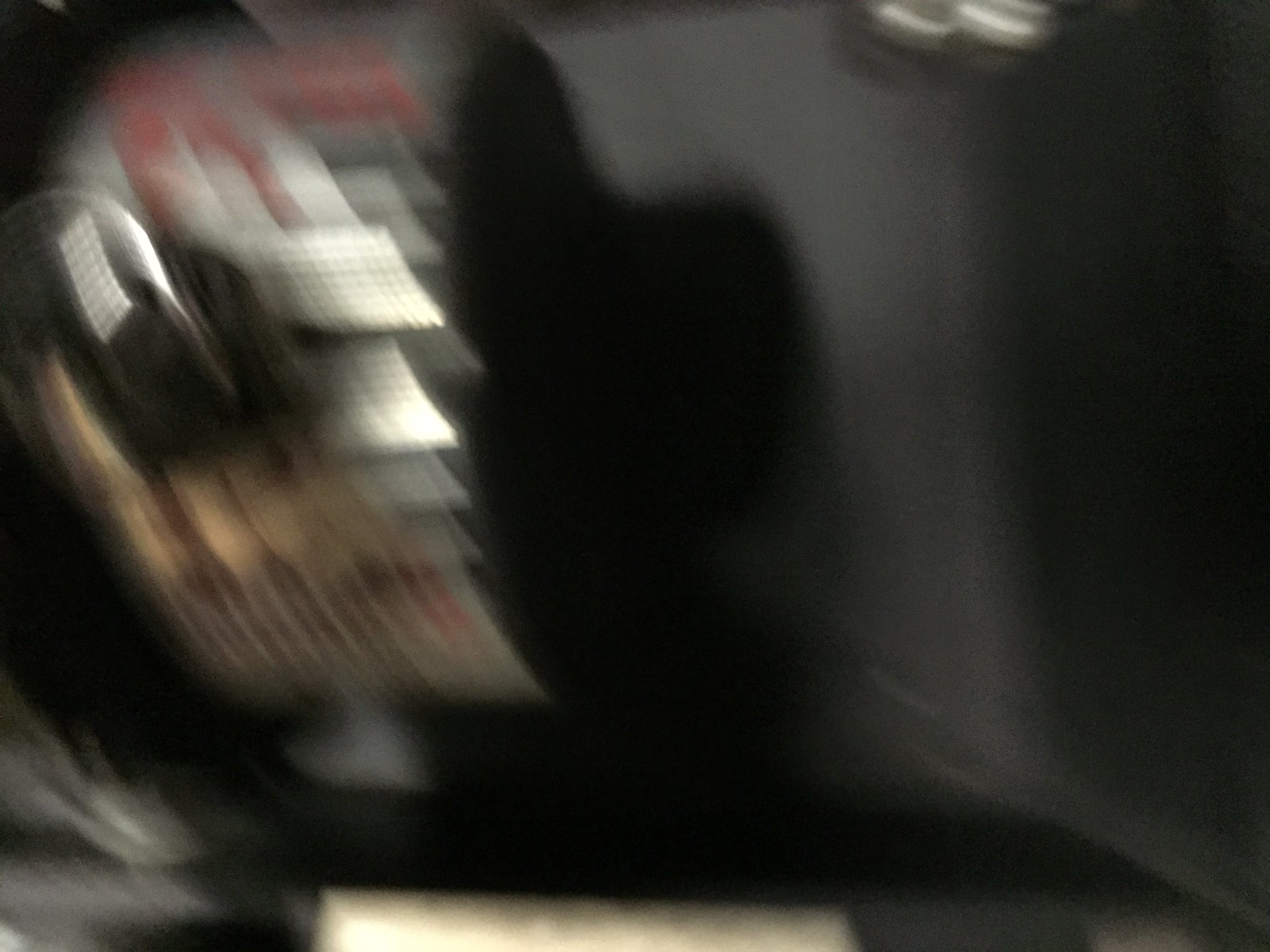A heavily blurred indoor photograph taken in low light conditions. The image lacks sharpness, making most features indistinct. On the left side, there are horizontal light streaks, transitioning from white at the top to tan and brown towards the bottom. These light streaks suggest illuminated panels, possibly from a car’s radio and temperature controls. In the center, a soft-edged black shape is visible, though its identity remains unclear. The right side shows a gray area, hinting at an interior vehicle surface. Additionally, a hint of something silver appears on the upper right edge, likely the car's dashboard vents. No text or other discernible details can be made out in the photograph.